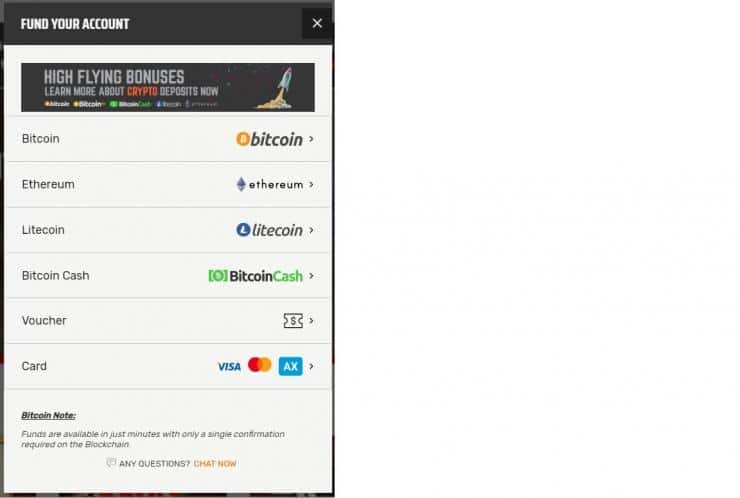A detailed image description of a mobile app interface focused on funding an account:

At the top of the screen, displayed on a mobile phone, there's a prominent deep brownish-colored rectangle featuring the text "Fund Your Account." On the right side of this rectangle, there is a darker brown circle containing a stark white "X" symbol, suggesting an option to close or exit the screen.

Just below this section, a highlighted advertisement banner promotes bonuses. It reads "High-Flying Bonuses: Learn More About Crypto Deposits Now," with the word "CRYPTO" distinctly emphasized in bold, all capitalized, orange letters, while the rest of the text remains in white.

Further down the screen, a list of cryptocurrency options is presented. Each currency name is positioned on the left, paired with an icon on the right:
1. "Bitcoin" is written in standard print. To the right, there's an elegantly designed text accompanied by a yellowish-orange Bitcoin icon.
2. "Ethereum" is listed next, with the text in regular print. Adjacent to it are two pyramid-shaped icons symbolizing Ethereum.
3. "Litecoin" follows, with "Lite" spelled as "L-I-T-E," and an associated icon.
4. "Bitcoin Cash" is listed similarly, followed by an icon.
5. "Voucher" is represented with a depiction of a coupon that appears to be torn, showcasing a dollar sign.

At the bottom of the screen, there is a section labeled "Card Area," which provides an interactive option allowing the user to choose their preferred payment method.

This detailed layout systematically guides the user through the process of funding their account using various cryptocurrency and payment options.